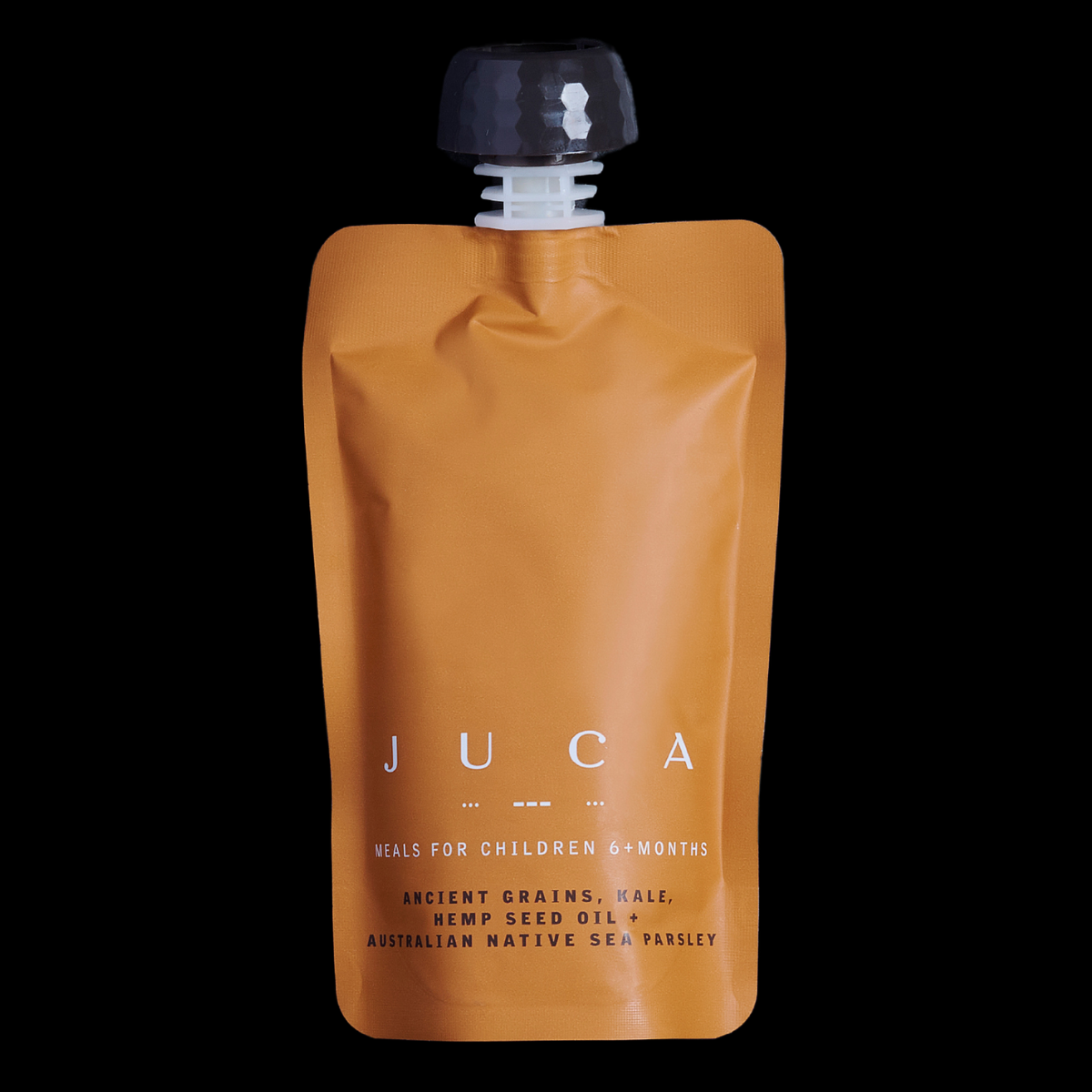This detailed photograph captures a close-up view of a child’s meal pouch, set against a stark black background. The pouch is primarily tangerine-colored with a subtle tan-gray hue and features a white neck tapering into a black, reflective plastic cap. The container, approximately five inches tall, appears filled with liquid and is likely designed for easy squeezing to dispense its contents. Prominently displayed on the pouch in clear text is "J-U-C-A," followed by the description, "Meals for children six plus months. Ancient grains. Kale. Hemp seed oil. Australian native sea parsley." The image is void of any human presence, focusing solely on the product in its simplistic, monochrome setting. The square format and absence of a border further emphasize the minimalistic and functional design of this nutritious meal option for young children.